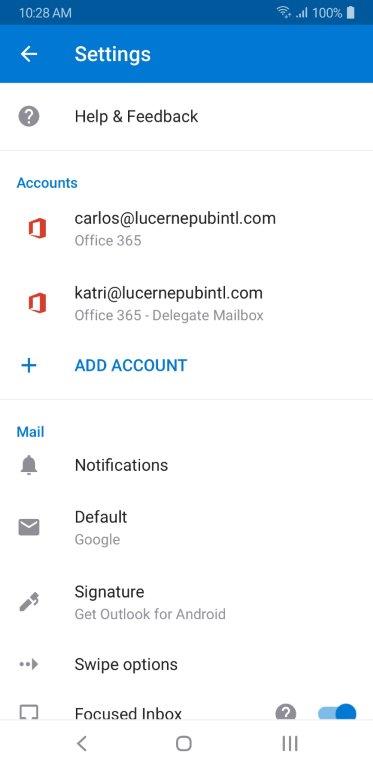The detailed descriptive caption of the image can be formulated as follows:

---

This is a colorful screenshot displaying a settings menu from a mobile phone. The top portion of the image features a blue band with a darker blue strip at the very top. On the upper left-hand corner within the blue strip, the time 10:28 AM is displayed in a blue font against the blue background. To the right, there are icons showing Wi-Fi connectivity and a fully charged battery at 100%.

Beneath the dark blue strip, the lighter blue band displays white text that reads "Settings" alongside a black arrow pointing to the left. Below this, the main body of the screenshot showcases a mostly white background with black text and various icons.

The first section is labeled "Help and Feedback," accompanied by a question mark icon. Following this, there is a section for "Accounts" highlighted in blue, listing two accounts: "Carlos at lucinapuntil.com, Office 365" and "Catrí at lucinapuntilint.com, Office 365, delegate mailbox." Next to each account, there are red Office 365 icons for visual indication.

Below the accounts section, a blue link labeled "Add Account" is displayed, separated by a thin horizontal line. Further down, another section labeled in blue—possibly "Mail"—is visible but not entirely clear. Additional settings options are listed, including "Notifications" represented by a black bell icon, "Defaults" featuring a Google envelope icon, "Signature" labeled as "Get Outlook for Android" with a pen icon, and "Swipe Options" with a right-facing arrow.

The "Focused Inbox" option includes a checkbox-like indicator (which might be unclear) accompanied by a question mark icon and a blue slider that is set to "on."

At the bottom of the image, there are navigation icons: a back arrow, a round home button, and three vertical lines representing the recent apps menu.

---